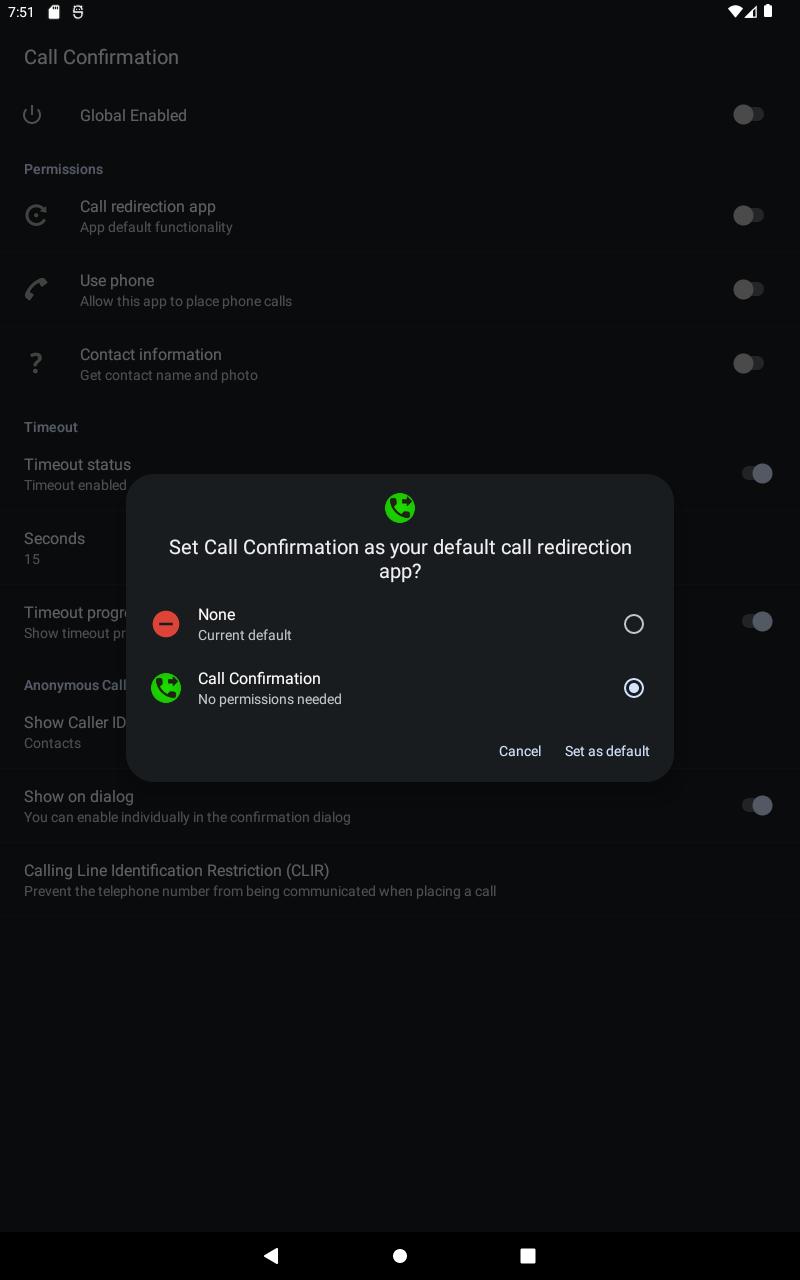Screenshot of Call Information Settings on a Mobile Device

The image is a screenshot with a black background and white font, depicting call information settings on a mobile device. 

In the top left corner, the time is displayed as 7:51, accompanied by two additional icons. The top right corner shows the signal strength indicators for both internet and phone connectivity, along with the battery level icon.

Below these indicators, the screen is divided into various sections:

1. **Global Settings**:
   - Label: "Global Enabled"
   - A toggle switch is available to turn this setting on or off.

2. **Permissions**:
   - **Call Redirection App**:
     - Label: "App default functionality"
     - A toggle switch allows the user to enable or disable this feature.
   - **Use Phone**:
     - Label: "Allow this app to place phone calls"
     - A toggle switch is provided for this permission.
   - **Contact Information**:
     - Label: "Get contact name and photo"
     - A toggle switch allows the user to enable or disable access to contact information.

3. **Timeout Options**:
   - **Timeout Status**:
     - Label: "Enable or Disabled"
     - Currently set to "Enabled".
     - Seconds: The timeout is set to 15 seconds.
   - **Timeout Program**:
     - Options include "Anonymous Call," "Show Caller ID," and "Show on Dialogue".

At the bottom of the screen, a pop-up box prompts the user to set the call confirmation as the default call redirection method, offering options for "None" or "Call Confirmation".